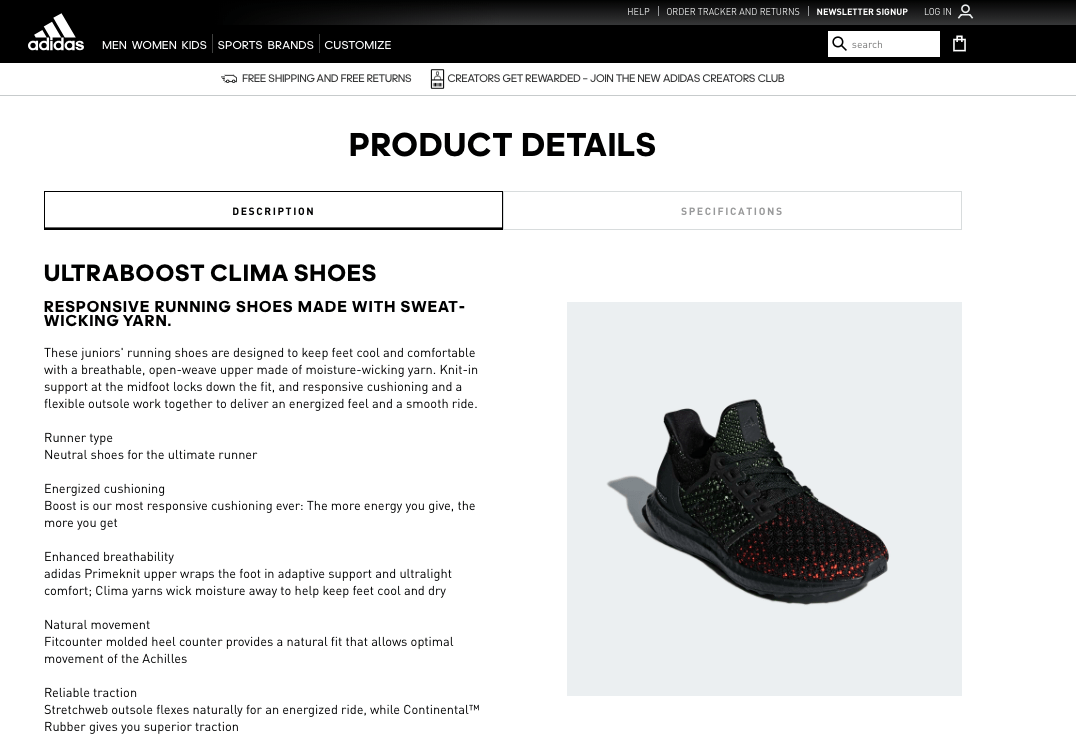The image appears to be a screenshot from the Adidas website. At the top, there's a dark black header. On the left side of this header, the iconic Adidas logo is featured, consisting of the brand name "adidas" in lowercase letters accompanied by three bars above it. To the right of the logo, a horizontal menu bar lists the options: Men, Women, Kids, Sports, Brands, and Customize. Extending to the far right side of this header, there is a white search bar with a black magnifying glass icon on its left.

Immediately below the header, on a clean white background, the bold capitalized text reads "PRODUCT DETAILS". On the right-hand side of the image, there is a detailed photograph of a single shoe. This shoe, identified as the Ultra Boost Klima Shoes, is primarily black with subtle red highlights at the front, visible through a mesh-like design. The shoe's toe is pointed towards the lower right corner, while the heel angles towards the upper left, casting a shadow that follows the same direction within a light gray square frame.

To the left of the shoe image, a rectangular box labeled "Description" contains details about the shoe. Below this header, the product name "Ultra Boost Klima Shoes" is prominently displayed, followed by a brief description stating, "Responsible running shoes made with sweat-wicking yarn." Further down, there are roughly twenty lines of detailed product information, segmented into various sections.

Adjacent to the "Description" box, another section titled "Specifications" appears in light gray text.

Between the black header at the top and the "Product Details" title, there is an icon of a truck. Next to this icon, two statements appear: "Free shipping and free returns" and "Creators get rewarded. Join the new Adidas Creators Club."